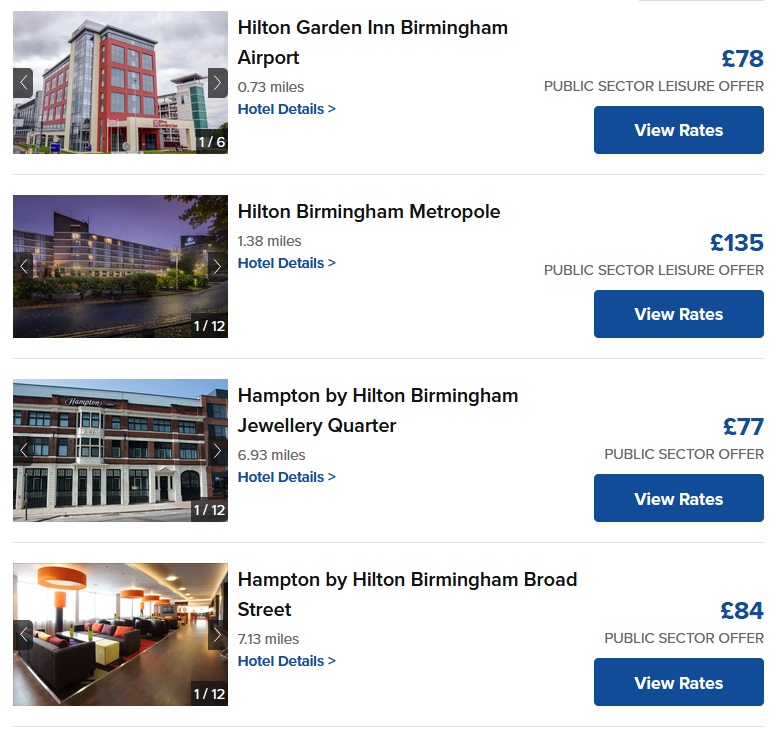Here is a cleaned-up and detailed caption for the image described:

---

This page from a travel website showcases four hotel listings with corresponding images and details. The background is white, featuring the hotel images on the left side. The hotel names are centrally positioned, while the rates and other pertinent information are aligned to the right.

1. **Hilton Garden Inn Birmingham Airport:**
   - Image Description: A four-story, red-brick hotel with numerous glass windows under a gray, cloudy sky.
   - Distance: 0.73 miles from the airport, indicated in gray text.
   - Details: "Hotel details" in smaller blue text.
   - Rate: £78, highlighted in blue.
   - Offer: "Public sector leisure offer" in gray text.
   - Action: A blue "View rates" button.

2. **Hilton Birmingham Metropole:**
   - Image Description: A nighttime view of a hotel characterized by extensive glass windows and balconies, facing a street.
   - Distance: 1.38 miles, shown in gray text.
   - Details: "Hotel details" in small blue text.
   - Rate: £135, highlighted in blue.
   - Offer: "Public sector leisure offer" in gray text.
   - Action: A blue "View rates" button.

3. **Hampton by Hilton Birmingham Jewellery Quarter:**
   - Image Description: A three-story building featuring a mix of brick and white façade.
   - Distance: 6.3 miles, indicated in gray text.
   - Details: "Hotel details" in smaller blue text.
   - Rate: £77, highlighted in blue.
   - Offer: "Public sector offer" in gray text.
   - Action: A blue "View rates" button.

4. **Hampton by Hilton Birmingham Broad Street:**
   - Image Description: An indoor view, likely a lobby or seating area, showcasing brown couches with red and brown pillows, yellow tables, and modern orange lights overhead.
   - Distance: 7.3 miles, shown in gray text.
   - Details: "Hotel details" in smaller blue text.
   - Rate: £84, highlighted in blue.
   - Offer: "Public sector offer" in gray text.
   - Action: A blue "View rates" button.

---

This detailed caption provides a clear and organized description of the travel website page, helping readers easily understand the contents and layout of the listings.